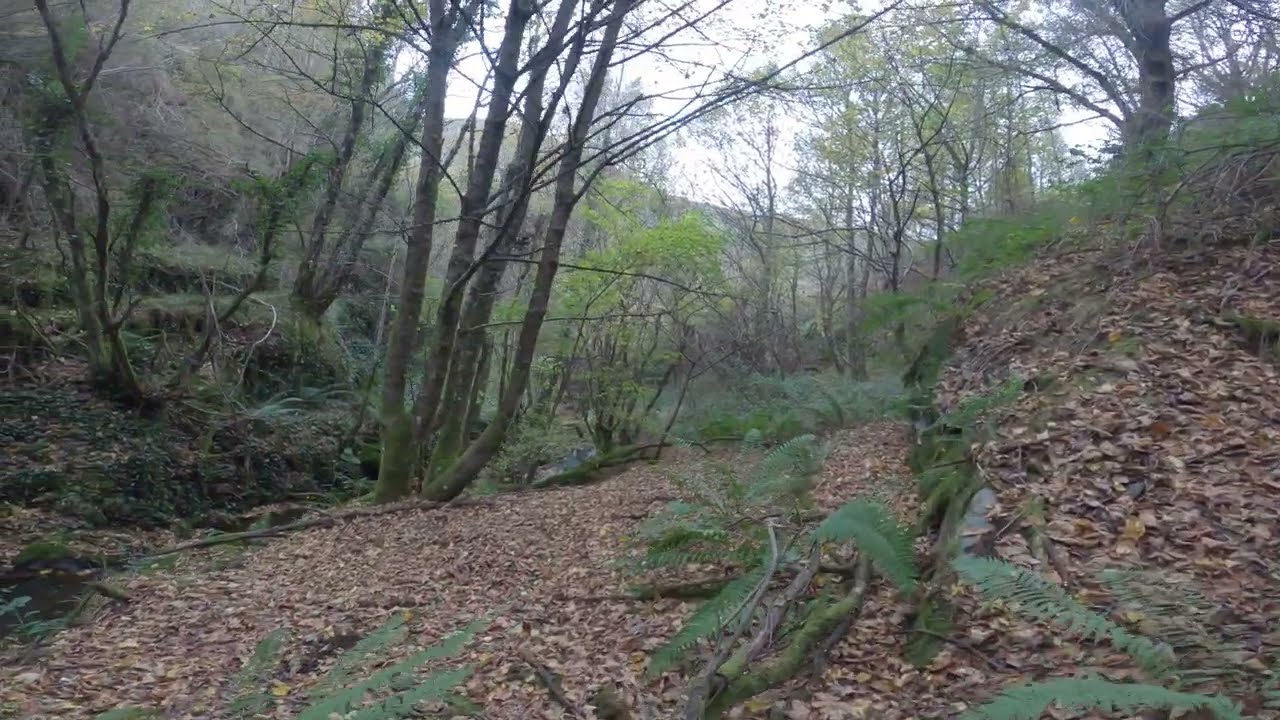This detailed photograph captures a serene forest scene bathed in natural daylight, evident from the predominantly white sky. The ground is carpeted with a mix of brown leaves and green fern plants, accompanied by twigs and small saplings emerging. The surrounding trees, which vary in size and height, display bark in shades of brown and gray, with many covered in patches of moss, lending a textured quality to the forest. In the background, the landscape subtly rises into hills or perhaps mountains, suggesting a distant elevated terrain. Centrally, faint hints of a small creek meander through the scene, enhancing the sense of tranquil wilderness. There are no people or animals visible, highlighting the untouched nature of this forested area. The overall composition of the image emphasizes the density and diversity of vegetation, with layers of leaves, ferns, and clusters of trees contributing to the lush, green ambiance.